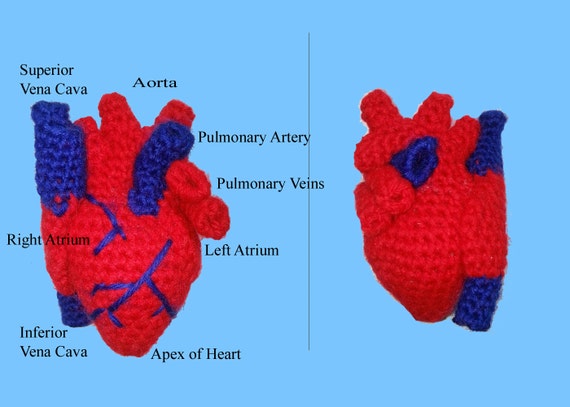The infographic features a realistic, anatomically accurate heart crafted from crocheted yarn, set against a light blue background. There are two distinct three-dimensional views of the heart. The image on the left provides an anterior view with detailed labels, indicating the superior vena cava, right atrium, inferior vena cava, apex of the heart, left atrium, pulmonary veins, pulmonary artery, and aorta. The heart is depicted using predominantly red yarn, with blue yarn highlighting specific arteries and compartments. The right image shows a side view of the same crocheted heart, rendered without labels, offering a contrasting perspective to the detailed depiction on the left.